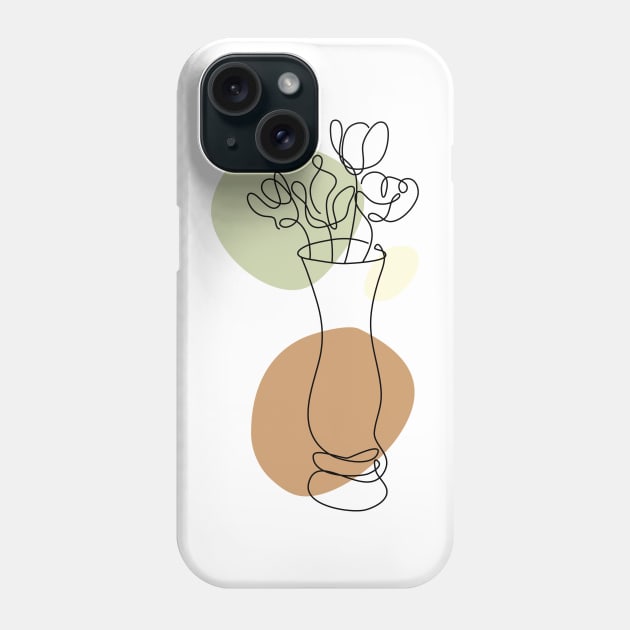This image depicts the back of a white iPhone case set against a gray background. The iPhone case features an artistic design centered around a tall vase with stemmed flowers, drawn abstractly using continuous black lines, giving it a holographic appearance. The design includes three distinct, overlapping circular shapes: a large brown circle at the bottom, a muted green circle near the top below the camera, and a smaller beige circle in between. The circles are transparent, allowing the intricate line drawing of the vase and flowers to be visible through them. The black iPhone camera, with its two large round lenses and additional smaller round components, is also prominently displayed at the top, adding to the detailed and artistic appeal of the phone case.